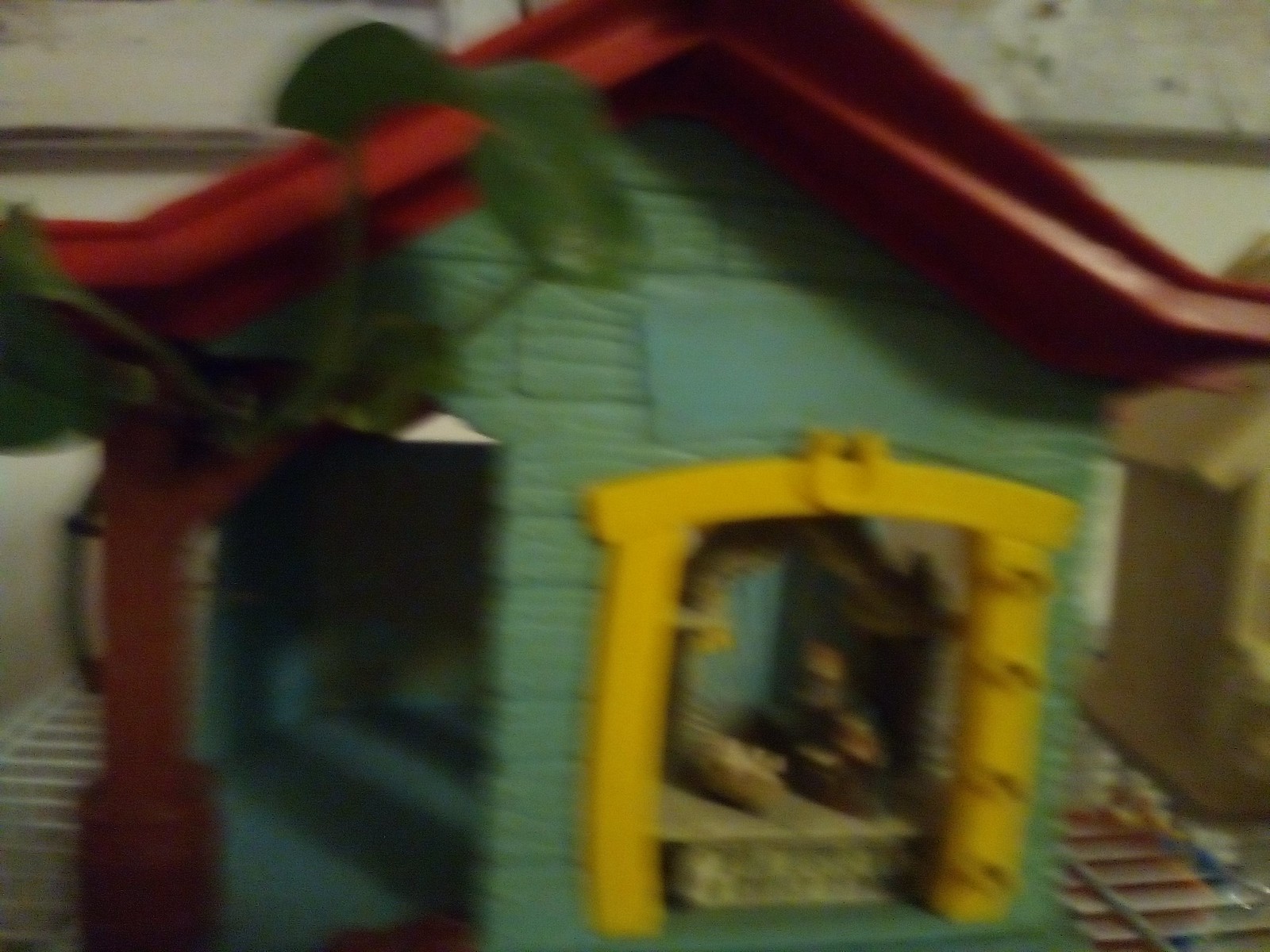The image depicts a close-up view of what appears to be a child's playhouse or toy house, captured in a somewhat blurry manner. The toy house is primarily made of green plastic and features a red roof. One of its windows is accented with medium yellow trim, which includes a yellow horseshoe-like detail above it. The playhouse sits adjacent to another structure, which appears to be a lighter wood-colored toy house. In the background, there's a tan-colored wooden panel or siding, alongside some visible leaves, indicating the presence of house plants. Inside the green toy house, there appears to be a large snake or a figurine, situated on what looks like a countertop. To the right side of the image, brown train tracks are partially visible, and the wall behind the setup is a whitish color.